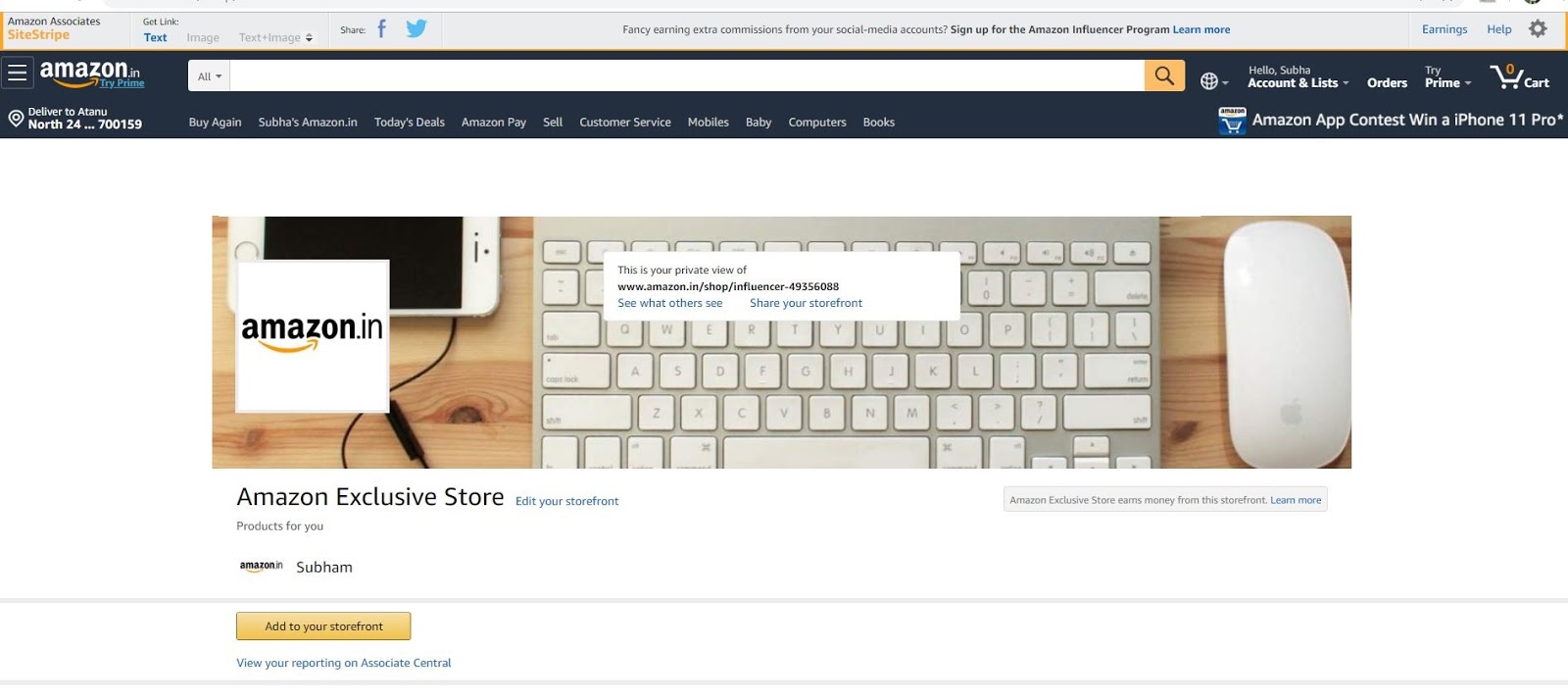The screenshot displays a computer screen with the official Amazon Exclusive Store website open. In the top-left corner, the recognizable Amazon logo is visible along with an indistinct "Deliver to" location, possibly beginning with "North 24," though the text appears unclear due to its small size. Centered on the webpage is a prominent search bar, and towards the top-right corner are various navigational options including "Account and Lists," "Orders," "Try Prime," and a shopping cart icon.

Beneath these elements is a promotional banner announcing an "Amazon app contest" with a chance to win an iPhone 11 Pro. The banner image is a wide rectangle featuring a sideways iPhone on the left side overlaid with an Amazon.in logo. To the right of the iPhone, there is an Apple keyboard and an Apple Magic Mouse positioned neatly.

Directly below this promotional image, the text denotes "Amazon Exclusive Store," followed by a series of instructional messages advising users to "Edit your content," and mentions the absence of a storefront with "No storefront," and an invitation to "Add to your storefront." Additionally, it advises users to conduct their reporting on "Associates Central."

The overall content and structure suggest this is a landing or setup page for building or managing an Amazon store, providing essential tools and information for store customization and reporting.